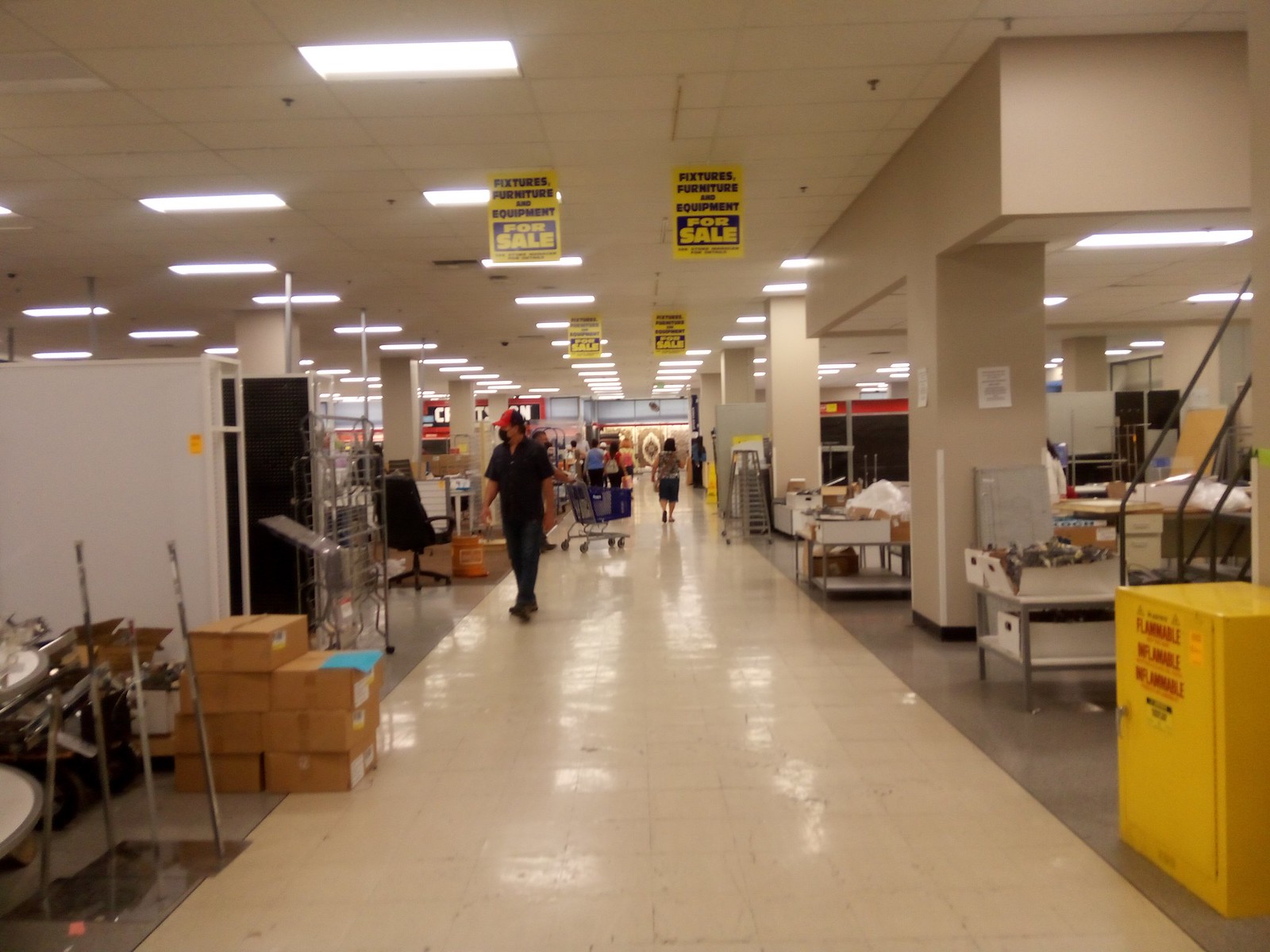This is a detailed color photograph taken indoors at a department store. The focus is on a large aisle with white tile flooring, accentuated by lighter gray linoleum along the edges. The ceiling features suspended fluorescent lights and yellow “For Sale” signs for fixtures, furniture, and equipment. The scene shows various items for sale, including shoes, microphone stands, and office equipment along the aisles, which appear somewhat messy with boxes haphazardly placed. On the bottom right, a stairway and a yellow box marked "flammable" are visible. Shoppers are seen navigating the aisle: a man wearing a red and black baseball hat, a face mask, a black shirt, blue jeans, and boots stands midway down; behind him is someone pushing a blue buggy; and off to the right, a lady in a skirt walks along. The store, despite signs of wear and disorganization, is active with people shopping.